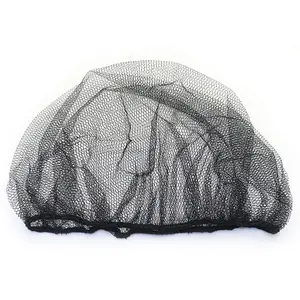The image features a black hairnet set against a stark white background. The hairnet has a semi-circular shape and appears mesh-like, composed of numerous intersecting lines and dots. It has an uneven, netted texture with visible cracks and lines that suggest an intricate weave. A thicker black band runs along the bottom edge of the hairnet, providing some structure to its otherwise delicate form. This detailed piece, commonly used by chefs and kitchen staff, exudes fragility and would likely collapse easily in the wind, adding to its ephemeral appearance.